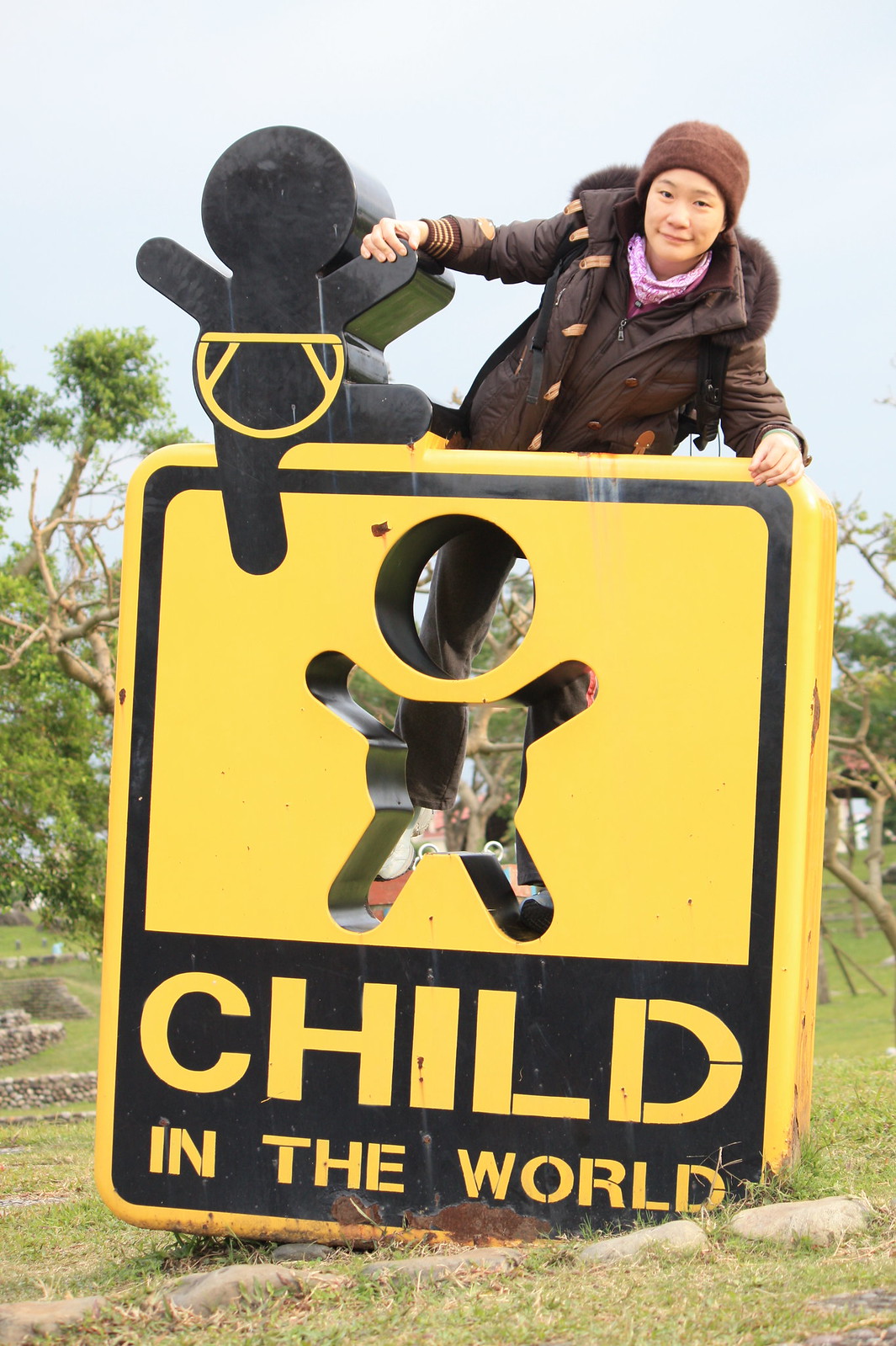In a remarkably vivid outdoor scene, set against a backdrop of grasslands and interspersed with trees, a prominent yellow and black sign stands out. The sign is rectangular with rounded corners and features a distinct depiction: on its yellow background, a black stick-figure child with a circular head and extended limbs is prominent. Directly beneath this figure, the sign transitions to a black color, bearing the inscription "CHILD IN THE WORLD" in bold yellow letters. Atop this sign is a young female, estimated to be around 20 years old, clad in a brown coat with yellow snaps, a matching knitted cap, and a pinkish scarf peeking out from underneath. She appears to be leaning over the top, interacting with the black cut-out figure of a child, which seems to have a yellow diaper-like detail. The composition is further enriched by a partly cloudy sky, the absence of other people, animals, or cars, and a mixture of blue, white, brown, yellow, and black colors that punctuate the overall picturesque scene.